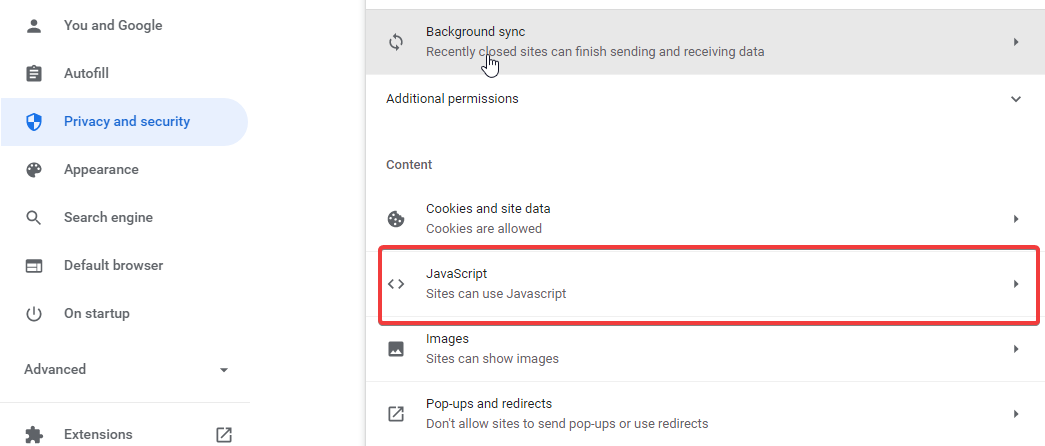The image depicts a detailed view of a laptop screen focusing on the "Privacy and security" section in a web browser settings menu. The overall background is white, and on the left side, about a third of the way over, there is a vertical column of setting categories.

In the top left corner, there is a profile icon next to the text "You and Google" in black. Just below, a section labeled "Autofill" is displayed alongside a small white-bordered square icon. The third section down is highlighted with a blue tab and features a blue and white shield icon with the text "Privacy and security" written in blue beside it, which is currently selected.

To the right of this highlighted section, there are four more icon sections labeled, including "Advanced" and "Extensions" located at the bottom of the left sidebar.

To the right of the sidebar is the main "Privacy and security" settings area, bordered by a gray vertical line on the left and topped with a gray rectangle. Inside this rectangle, a refresh icon is situated on the left, followed by the text "Background sync" in black. Beneath this, a description reads "Recently closed sites can finish sending and receiving data," next to a hand-pointing icon.

Below the gray rectangle, the area transitions to a white background, displaying the heading "Additional permissions" in black. Underneath this, there is a section labeled "Content" featuring four options, each represented by icons on the left and names on the right. The second option, "JavaScript," is highlighted with a blue rectangular border, indicating it is selected for further settings adjustment.